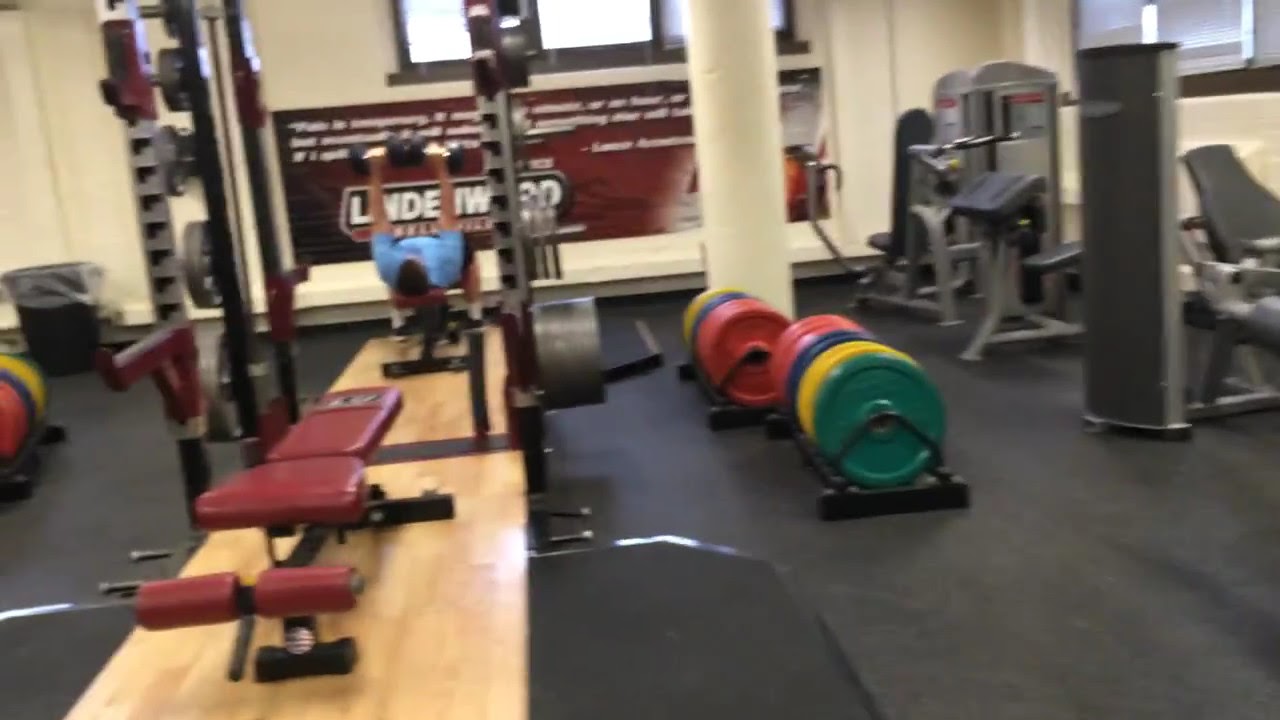In this detailed gym scene, the focus is on a solitary person in a blue t-shirt, lying prone on a bench and lifting weights. The individual’s feet are firmly planted on the ground while their hands extend above, moving the weights up and down in a rhythmic motion. The gym is devoid of other people, emphasizing the sense of solitude in the workout. Various weight plates in vibrant colors—green, blue, yellow, and red—are scattered in the background, along with an assortment of gym equipment including benches, a bench press machine, a leg exercise machine, a pull-up machine, and a bicycle. The setting seems to capture just a section of the larger gym, with a partial view of a sign in the background that reads "LINDWORD LINDWORD."